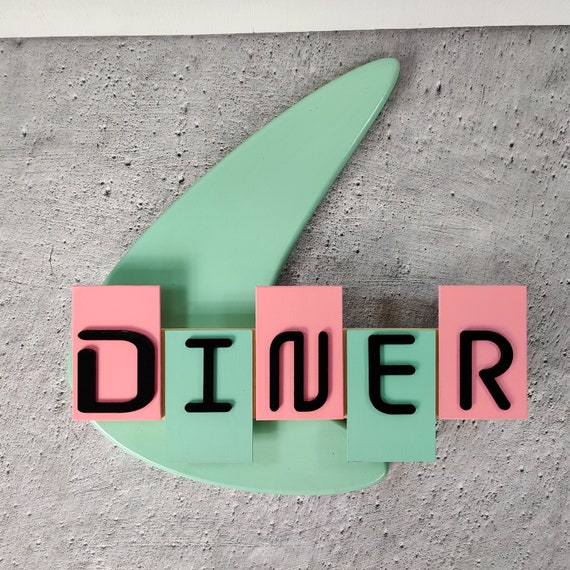The image is square-shaped and features a close-up of a retro-style diner sign attached to a light gray, porous stone wall. The background of the sign includes a vertically mounted, mint green boomerang-style swoosh. The word 'Diner' is spelled out in black letters, each on a separate rectangle that alternates in color and height atop the swoosh. The first rectangle, holding the letter 'D', is light pink and positioned higher than the rest. Next is a green rectangle with the letter 'I', placed slightly lower. This pattern continues with a pink rectangle for 'N', a green rectangle for 'E', and finally, a pink rectangle for 'R', all creating a vibrant, staggered effect while the word itself remains level.